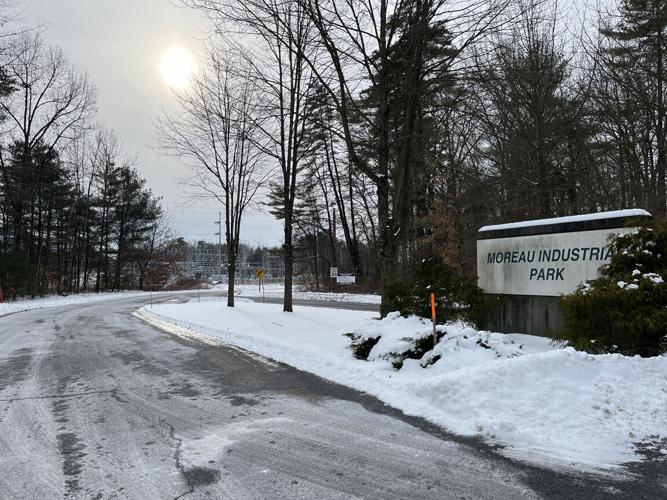The photograph, an outdoor daytime shot, is rectangular, measuring roughly five inches wide by four inches high. It captures a scene centered around a road, which starts in the lower right-hand corner, curves leftward, then doubles back toward the right-center of the image. The road is clear but shows signs of recent ice, with plowed snow gathered along the edges. Prominently featured on the right side of the road is a snow-covered median, home to a large stone sign that reads "Moreau Industrial Park." Flanking this sign are several deciduous trees, bare of leaves, and a nearby stake marked with orange. In the background, both deciduous and evergreen trees are visible, with a clustering of power grids and structures indicative of a power plant further down the road. A diamond-shaped sign at the road's end, displaying an arrow, warns of a sharp right turn. Overhead, the sky is gray, with the sun, a bright white circle outlined in orange, prominently positioned in the upper left-hand corner.